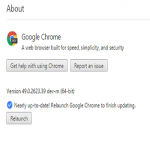A small, somewhat blurry screenshot showcasing a notification screen, possibly taken from a computer. At the top left, the word "About" is visible, followed by "Google Chrome." Below this, the phrase "a web browser built for speed, simplicity, and security" appears, though it’s difficult to read clearly. There are two buttons beneath the text: one on the left labeled "Get help with using Chrome" and another on the right labeled "Report an issue." Just below these buttons, a version number is shown, but it is illegible in the screenshot. Additionally, another notice is present, along with a "Relaunch" button at the bottom.